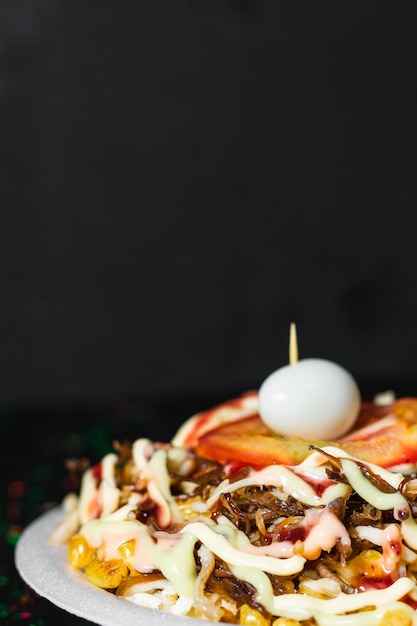This close-up image focuses on a partially visible white styrofoam plate positioned in the bottom right corner against a black background. The plate features a diverse assortment of foods, making the dish somewhat ambiguous. Visible items include corn, slightly melted cheese strands, and well-cooked beef and onions, suggesting a hearty meal. Among the toppings, there is a red bell pepper or tomato slice and a hard-boiled egg secured with a toothpick. Additionally, there are two distinct sauces—one greenish and one pinkish—adding to the array of colors and textures. The scene is softly illuminated by dim, distant lights resembling Christmas lights in the bottom left, enhancing the detailed and appetizing presentation of the food.